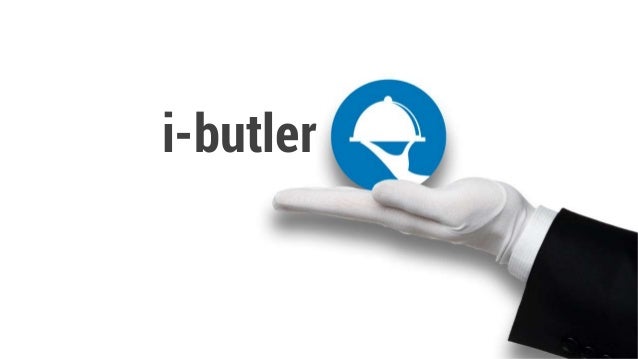The image is a digitally edited graphic combining photography and software enhancements. Set against a pure white background, a hand wearing a pristine white glove extends from the bottom right corner. The hand, emerging from a black-sleeved arm suggesting a formal suit, lays flat as if presenting something. On top of the gloved hand rests a blue circle with a white stylized image resembling a butler's serving dish. The glove, tight and slightly wrinkled near the wrist, reveals some fingernail contours, emphasizing its elegant, close-fitting nature. To the left of the blue circle, in black text, the word "i-Butler" is clearly displayed, suggesting this is likely a promotional image for an app named iButler. The overall composition is simple yet distinct, exuding class and sophistication.